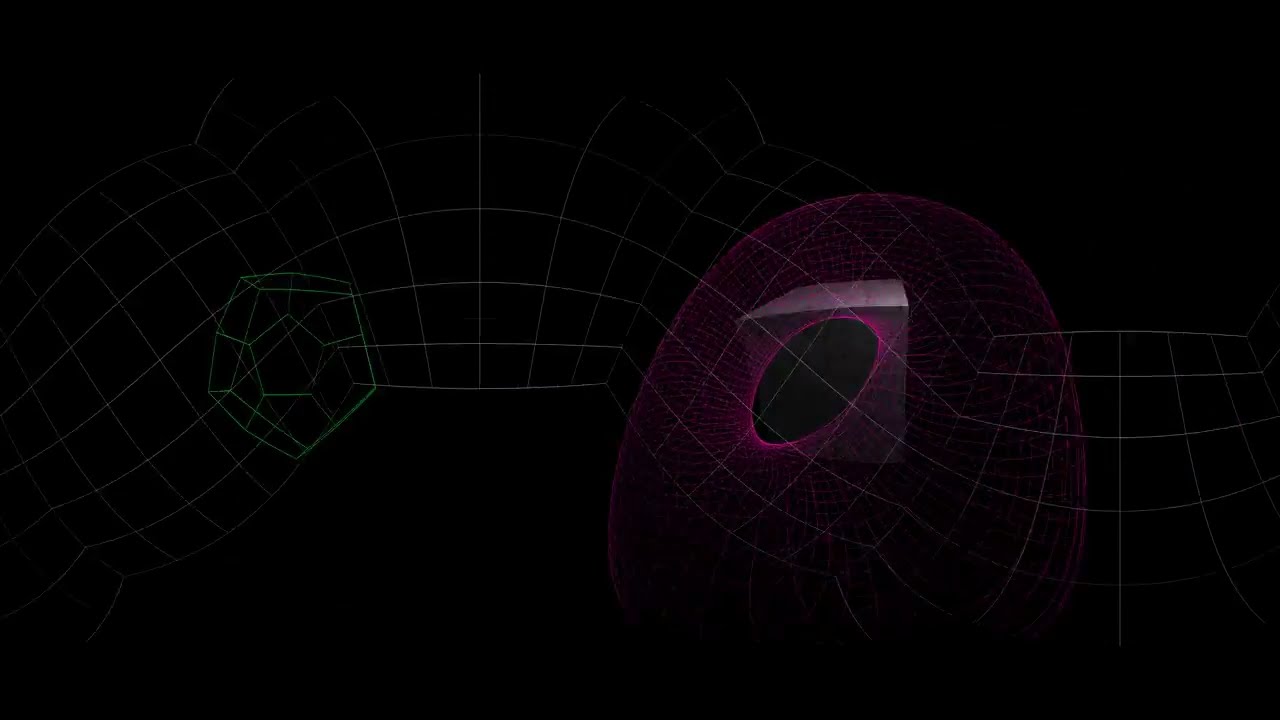The image is set against a completely black background and features a digitally created, geometric design stretching across the entire center. The design consists of various mathematical curves, patterns, and shapes, including structures that look like interlocking green pentagons forming a nearly circular shape and red, sweeping half-circle lines. These elements are arranged over a white grid and give the appearance of being three-dimensional, with some of the lines creating a 3D effect akin to humps protruding outward. Additionally, there's a pixelated, checkered pattern in purple and black, and a shape resembling a soccer ball on the leftmost hump, characterized by its octagonal facets. The image is devoid of any text, emphasizing its abstract and artistic nature.